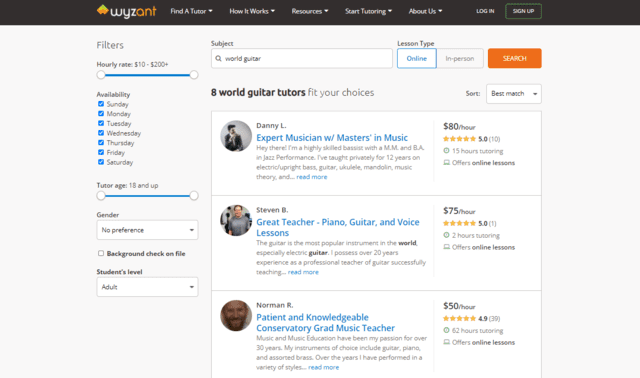Screenshot of the Wyzant Tutoring Website:

The screenshot captures the homepage of Wyzant, a comprehensive tutoring platform, with the image oriented wider than it is tall. The background of the page features a subtle gray hue. Dominating the top section is a prominent black banner where, on the left side, the Wyzant logo is displayed. The logo creatively highlights "W-Y-Z" in white font and "A-N-T" in vibrant orange.

The banner also incorporates several dropdown menus labeled: "Find a Tutor," "How It Works," "Resources," "Smart Tutoring," and "About Us." Additionally, options to log in or sign up are available on the right side of the banner.

Focusing on the search functionality depicted in the image, the user appears to be seeking a guitar tutor. They entered "World Guitar" under the "Subject" field. The user's search parameters are quite broad, encompassing availability for all days, an hourly rate ranging from $10 to $200+, and a minimum tutor age of 18 with no upper limit. There is no gender preference specified, and the student level is set to "adult."

Based on these criteria, Wyzant has returned a list of eight tutors, as indicated by the message "8 World Guitar tutors fit your choices." Displayed within a white box below this message are the details of the first three tutors:

1. **Danny L.** - Headlined as an "Expert Musician with a Master's in Music," Danny charges $80 an hour.
2. **Steven B.** - Describes himself as a "Great teacher" specializing in piano, guitar, and voice lessons with an hourly rate of $75.
3. **Norman R.** - Touted as a "Patient and knowledgeable conservatory grad music teacher," Norman offers his services at $50 per hour.

This meticulous setup provides the user with a clear and detailed overview of available tutoring options for learning the guitar.